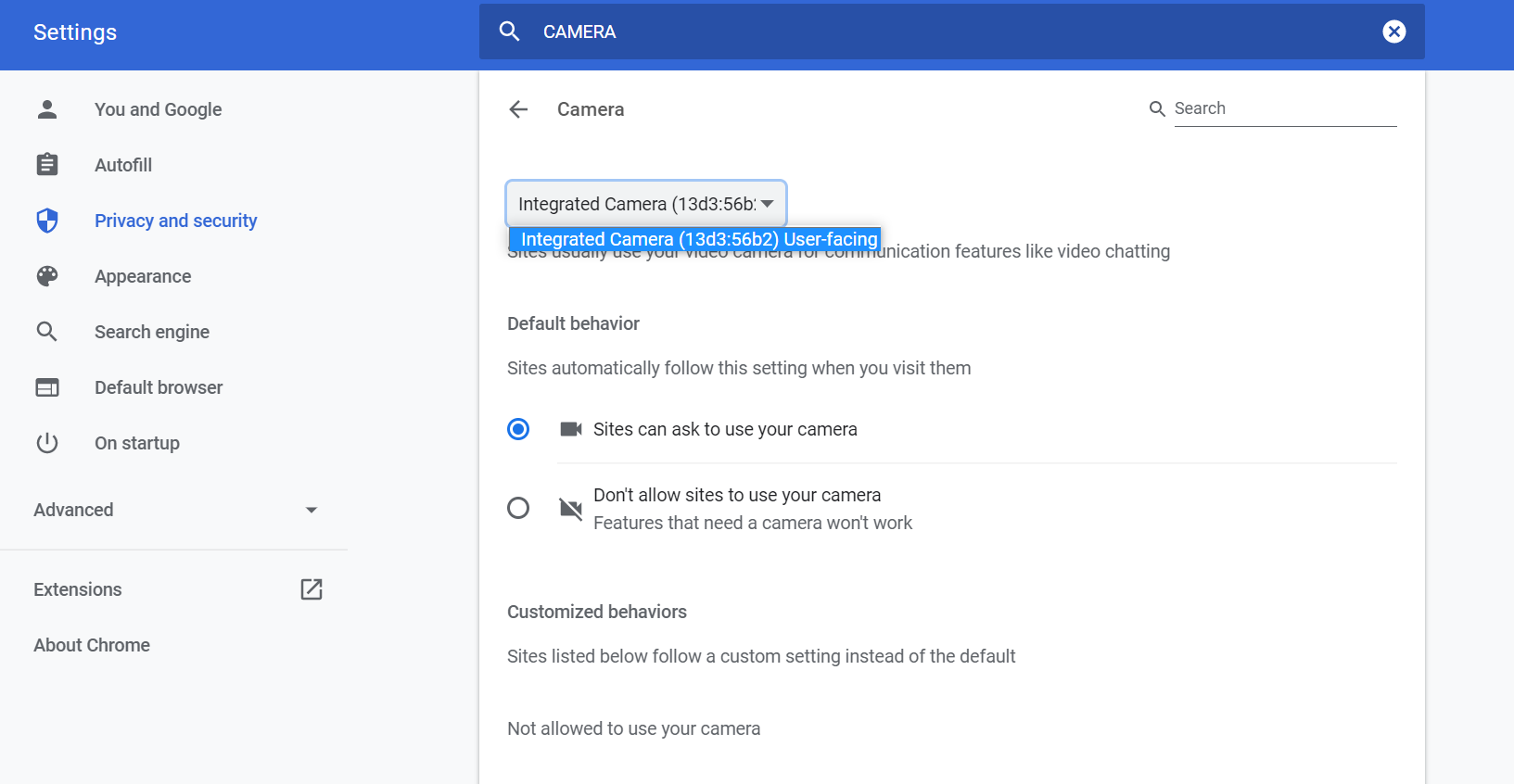Detailed Camera Settings Menu Description in Google Chrome:

In the provided image, a settings menu for the camera is displayed, which appears to belong to Google Chrome. The interface has a distinctly Windows-like appearance. 

At the top, there's a blue bar labeled "Settings." Below this bar, the word "Settings" is prominently displayed in white, contrasting with other black text.

The menu options include:
- **You and Google**
- **Autofill**
- **Privacy and Security**: This is highlighted with a clickable blue button.
- **Appearance**
- **Search Engine**
- **Default Browser**
- **On Startup**
- **Advanced**: This comes with a drop-down menu.

There is also a section for **Extensions** with an option to maximize the view and another section titled **About Chrome**.

Focused on the camera settings, the menu displays a back button and a search option. The heading "Integrated Camera" is followed by a device identifier, potentially "13D3:56B".

A pull-down menu is available for selecting camera options featuring labels like "Integrated Camera" and "User-Facing."

The menu outlines default behaviors for camera usage on websites:
- **Sites can automatically follow their settings**
- **Sites can ask to use your camera**

There are options to:
1. **Block sites from using the camera**, warning that features requiring the camera won’t work.
2. **Customize behaviors** for specific sites, visible in a list below with "custom settings" and options set to either default or not allowed to use the camera.

This comprehensive view makes it clear that these are Google Chrome settings focused on managing camera usage permissions.